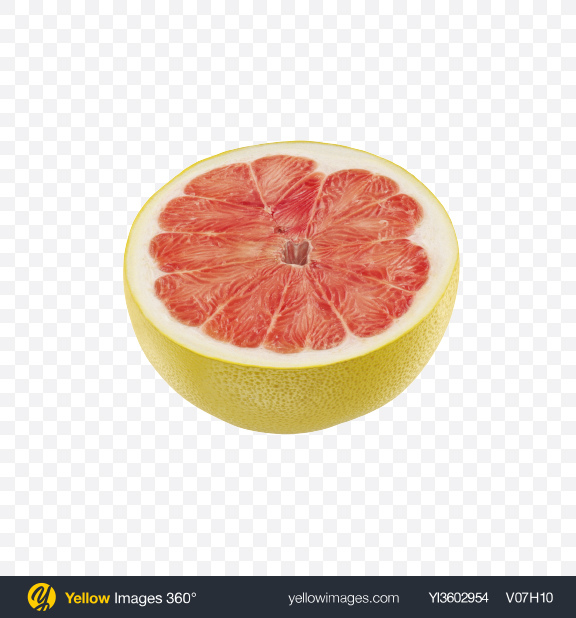This image showcases a stock photo of a halved grapefruit placed against a light gray and white checkered background. The grapefruit, with its top perfectly sliced off to form a flat surface, reveals an intricate inner structure resembling flower petals. The segments, arranged in a circular pattern, are a vibrant mix of bright pink and red hues, suggesting it is a ruby red grapefruit. These fleshy segments are encased by a white rind, and their triangular or heart-shaped forms culminate in a small central void. The exterior peel of the grapefruit features a textured appearance with speckled dots, displaying a blend of yellow with hints of greenish-orange. At the bottom of the image, there are text details: on the left-hand side, it reads "Yellow Images 360 degrees" accompanied by a Y logo, and on the right, it has the identifier "Y13602954" along with "V07H10."